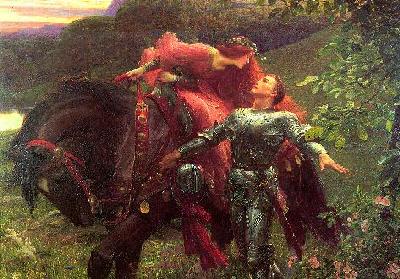The image showcases a classic, rectangular oil painting that exudes a fairytale-like, romantic atmosphere. A woman with long red hair adorned with a floral wreath rides a richly decorated brown horse, dressed in an elegant, floor-length red gown. She leans over to her left, gazing tenderly at a knight in armor standing beside the horse. The knight, characterized by his brown hair and outstretched arms, holds his helmet in his right hand, positioning as if about to share a kiss with the woman. The intricate details of the horse's bit and bridle add to the lavishness of the scene. The background depicts a dreamy landscape of mountains and a lake, bathed in the soft hues of a yellow and pink sunset. To the right, tree leaves frame the romantic tableau, contributing to the serene natural setting. The ground below features foliage, completing the picturesque and timeless scene.